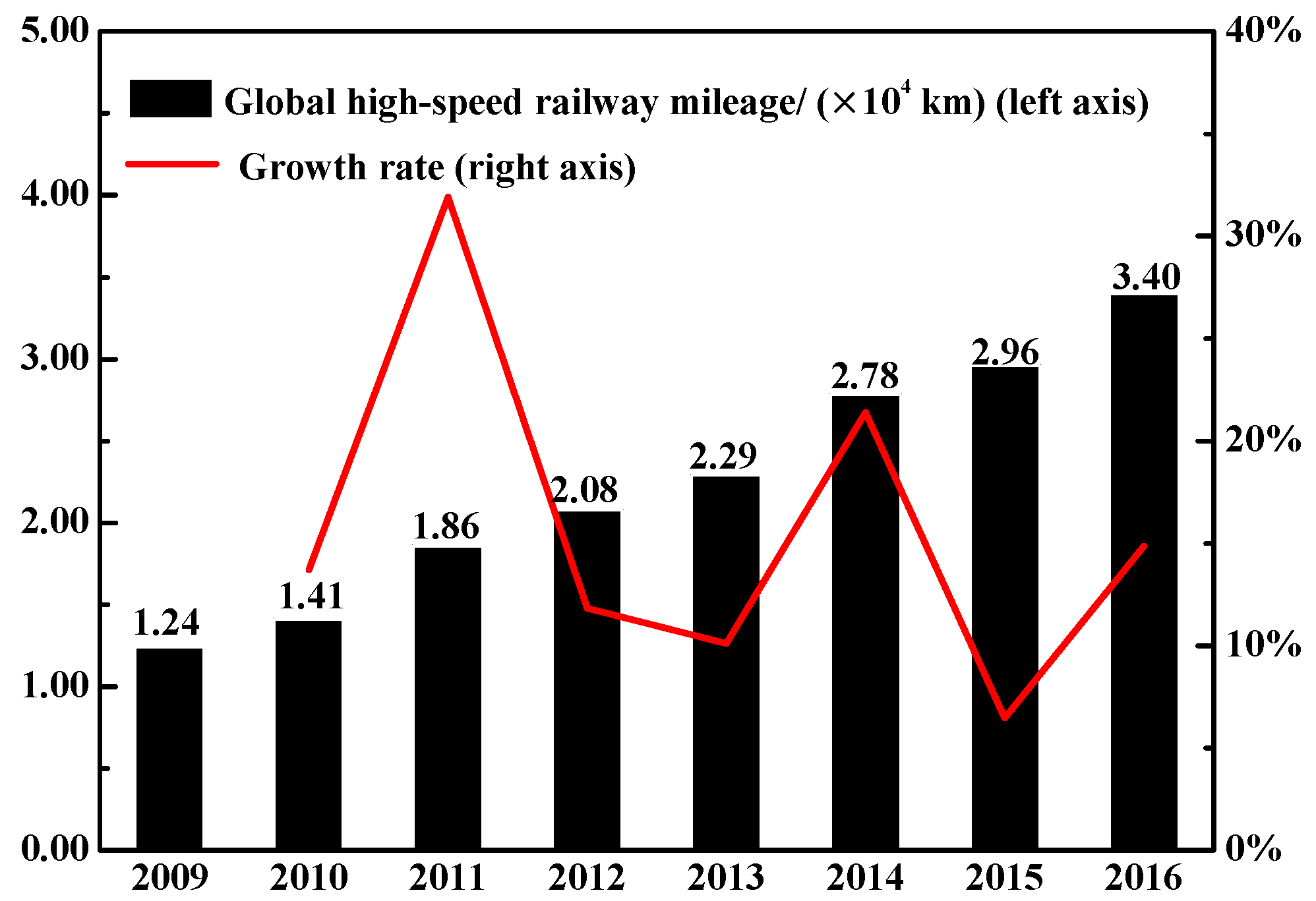The image is an Excel-generated combination bar and line graph illustrating global high-speed railway mileage and its growth rate from 2009 to 2016. The x-axis displays the years consecutively from 2009 to 2016. The left y-axis, labeled in kilometers and ranging from 0.00 to 5.00 in single integer increments, corresponds to the black bars on the graph. These bars represent the global high-speed railway mileage times 10 to the 4th power kilometers, showing a year-on-year increase: 1.24 in 2009, 1.41 in 2010, 1.86 in 2011, 2.08 in 2012, 2.29 in 2013, 2.78 in 2014, 2.96 in 2015, and 3.40 in 2016.

The right y-axis, ranging from 0% to 40% in increments of 10%, is tied to the red line graph representing the growth rate. The data for the growth rate starts in 2010 at approximately 15%, spikes to 30% in 2011, then drops significantly to above 10% in 2012. This downward trend continues slightly in 2013 before rising to around 20% in 2014. Thereafter, the growth rate plummets to 7% in 2015 and rebounds to 15% in 2016. 

The graph's legend at the top clarifies that black bars indicate global high-speed railway mileage, while the red line signifies the growth rate. The overall presentation is clear and well-lit, making it easy to read and interpret the data trends over the observed period.